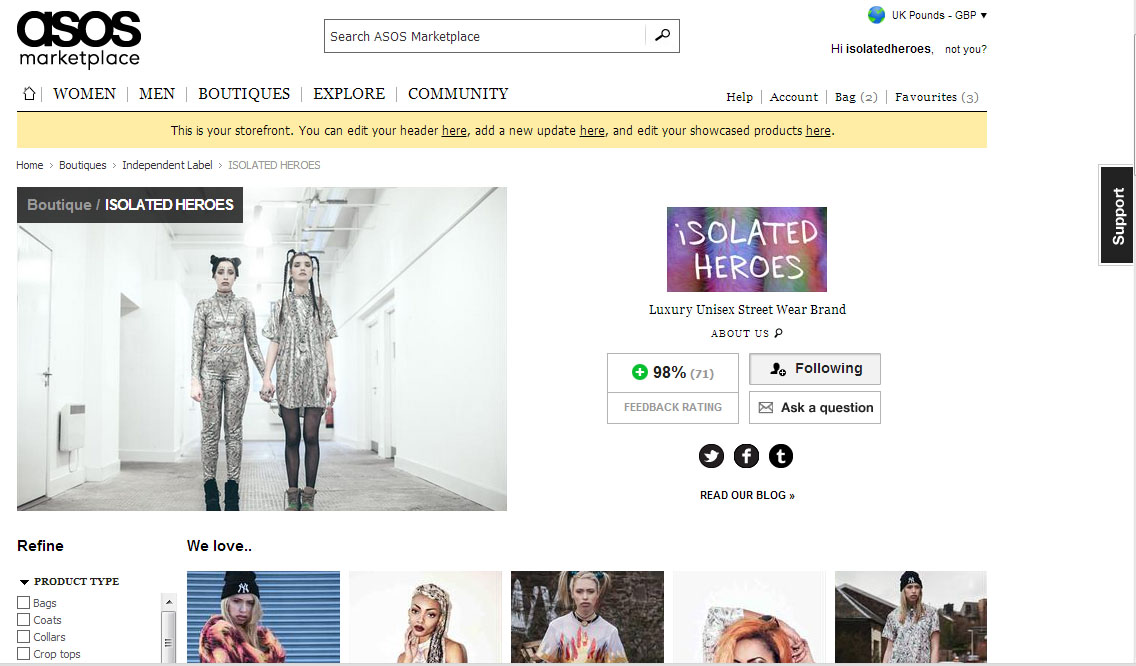Detailed Description: 

The image showcases a web page from the ASOS Marketplace, featuring a white background adorned with a subtle, thin gray border along the right and bottom edges, leaving the left and top edges seamlessly blending into the surrounding space. 

At the upper left corner, the ASOS logo is prominently displayed in bold, black font, with the word "marketplace" written underneath in a smaller font size. Just to the right of this, there is a search bar encased in a gray rectangular box, complete with a magnifying glass icon on the far right, indicating the functionality of a search tool.

Beneath this section, a navigation menu spans horizontally across the width. The menu items, namely Home, Women, Men, Boutiques, Explore, and Community, are displayed in capital letters. To the right of these, in a smaller, non-capitalized font, are additional links: Help, Account, and Bag, with parentheses noting two items under "Favorites" and three items under "Bag."

Below the main menu, a narrow yellow banner catches the eye, presenting a message for users managing their store. The banner reads, "This is your store storefront. You can edit your header here, add a new update here, and edit your showcase products here." The term “here” in each instance is underlined, indicating clickable links for further actions.

Further down, we observe breadcrumb navigation, which maps the user's journey within the site. It shows the pathway from Home to Boutiques, then to Independent Label, and finally to the current page labeled "Isolated Heroes," reflecting the specific boutique or label being viewed.

The layout and the positioning of each element reiterate a structured and user-friendly web interface, reflective of ASOS’s online marketplace.